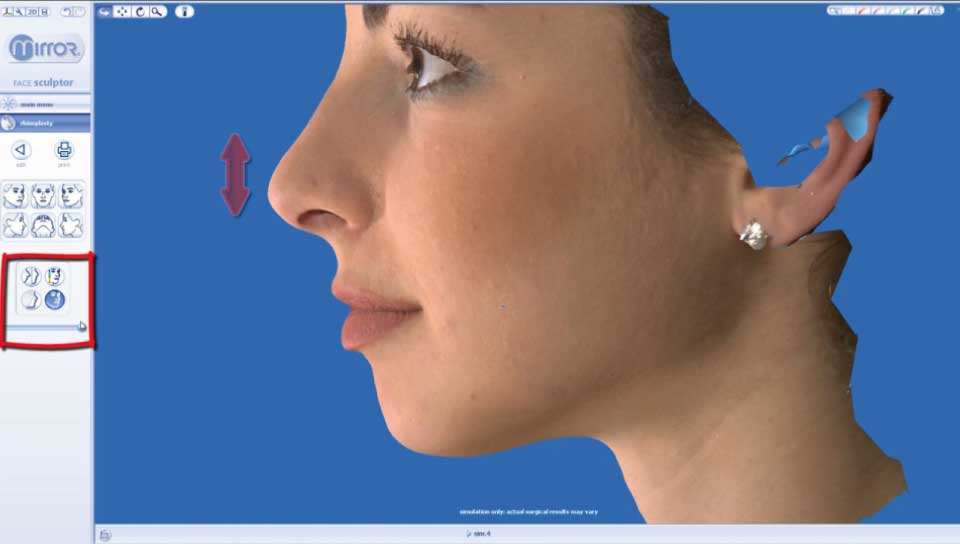The image appears to be a screenshot from a facial editing or reconstruction program, likely named "Mirror" as indicated by the trademarked label in the upper left-hand corner. The main portion of the screen features a blue background with the profile of a woman's face, centered with her head cropped at the top and back, leaving only a small portion of hair visible near her ear adorned with an earring. The woman, with a prominent nose, is facing toward the left of the viewer. An up-down arrow is placed in front of her nose over the blue background, hinting at adjustable features. Along the left side of the screen, there's a thin vertical bar presenting various face modification options, including multiple images showing different facial perspectives and a sculpting tool. Additionally, some blurred commands are visible at the top right of the interface, and a magnifying glass icon along with other buttons can be seen at the top left of the photo area.